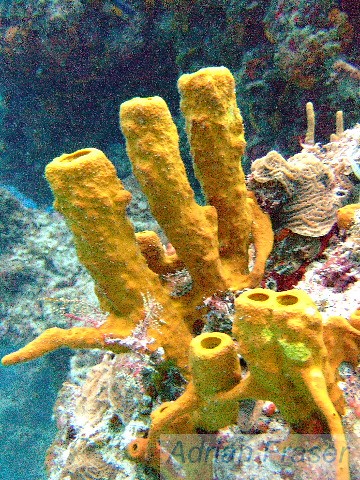This photo, likely taken with an underwater camera, showcases a vibrant and meticulously arranged aquarium scene. The central focus is a cluster of artificial sea anemones with tall, tube-like structures in shades of yellowish-orange, resembling stalagmites. These anemones are accompanied by shorter ones of the same type, creating a layered effect. Surrounding the anemones are various rocky, mountainous decorations, reminiscent of those found in pet stores for aquariums. The rocks display a mix of beige, jade, and rust colors, with some areas covered in moss. In the background, the clear blue water provides a serene backdrop to the scene, which also includes darker rocks, some with small growths, and a cave-like opening for fish to swim through. The name "Adrian Fraser" is prominently displayed in the bottom right-hand corner in black text within a white, faded rectangular box, indicating the photographer.